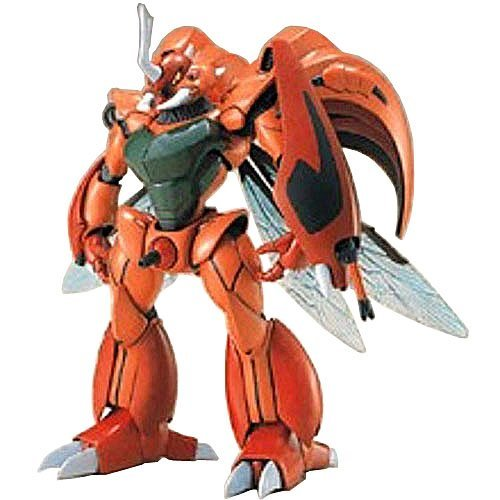This detailed caption brings out the shared features and emphasizes the unique aspects of the image described by both speakers:

The photograph appears to depict an intriguing action figure, possibly representing an alien monster robot. The figure sports a distinctive blend of orange, black, and white colors, reminiscent of a dragonfly or a ladybug. Its body is predominantly orange with stark black accents, and it features white elements on the wings, talons, and pincers-like fangs near its mouth.

Prominent wings extend from its back, suggesting the capability of flight, adding to the complexity of its design. Its humanoid form contrasts with insect-like attributes, such as sharp claws and small horns near the face, presenting a fusion of robotic and biological elements. With a black core and striking white details, the figure stands out, exuding a sense of strength and mechanical sophistication. Overall, this detailed action figure or computer-generated image highlights an inventive blend of creature and machine aesthetics, making it a fascinating piece.